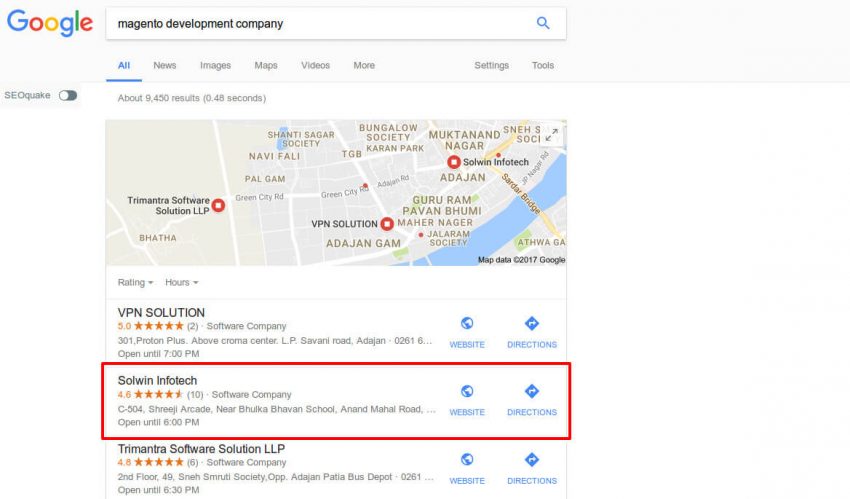The upper left corner of the image features the Google logo, consisting of a blue "G", red "O", yellow "O", lowercase blue "g", green "l", and lowercase red "e." Inside the search bar, the text "MAGENTO development company" is prominently displayed. Below the search bar, a navigation bar includes the categories "All" (highlighted in blue and underlined), "News," "Images," "Maps," "Videos," "More," "Settings," and "Tools". 

Directly beneath this navigation bar, the search results indicate "About 9,450 results in 0.48 seconds." The main content area features a map, with a blue line representing a body of water. Various business locations are marked with red circles on the map, including "Bungalow Society," "Solwin Infotech," "VPN Solution," and "TriMetra Software Solution LLP."

Below the map, specific business listings are detailed further:

- **VPN Solution**: Rated five stars, categorized as a software company.
- **Solwin Infotech**: Displayed in a red box, rated 4.6 out of 5 stars.
- **TriMetra Software Solution LLP**: Rated 4.6 out of 5 stars.

Each listing provides information pertinent to companies specializing in Magento development services.